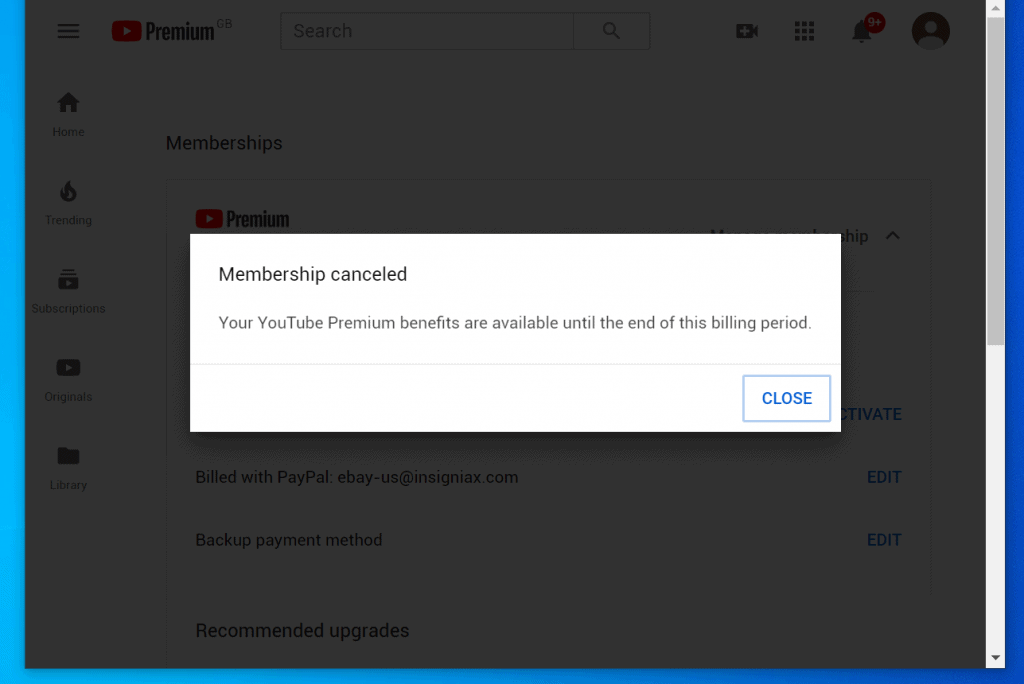A detailed screenshot of a YouTube Premium desktop interface, showcasing the cancellation of a membership. Dominating the screen is a white rectangular pop-up message that says, "Membership canceled. Your YouTube Premium benefits are available until the end of this billing period," with a "Close" button beneath it. This pop-up grays out the background, focusing attention on the notification.

At the top left corner, the YouTube logo is prominently displayed, followed by the word "Premium," confirming the user is on the YouTube Premium page. Beside the logo is a search bar, and further right, a row of four icons. From left to right, they include: a video camera icon, a grid icon composed of nine small squares, a bell icon with a red badge indicating "9+" notifications, and a profile icon depicting a simplistic human figure.

On the left sidebar, vertically aligned icons and text labels indicate major navigation sections: "Home" with a house icon, "Trending" with a fire icon, "Subscriptions" and "Originals" both represented by play button icons, and "Library" marked by a file icon. Visible below these are partial labels and icons, such as "Memberships" and "YouTube Premium", partially obscured by the pop-up.

In the partially obscured content under the pop-up, there is a visible text that reads "Build with PayPal, eBay, US at insigniax.com," followed by "Backup payment method." Below this, the phrase "Recommended upgrades" appears, each accompanied by an "Edit" option for modifications.